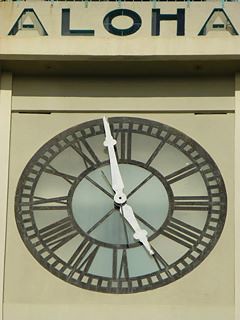The image portrays the side of an establishment, presumably located in Hawaii. Prominently featured is the word "Aloha" in bold, uppercase letters (A-L-O-H-A), situated above a classic clock with Roman numerals. The clock, with its white, pointed hands, suggests ease of readability. The background against which "Aloha" and the clock are set is a tan, cement-like texture, indicating that they are affixed to the exterior of the building. The angle of the sun implies a shiny surface on the clock, adding a reflective quality to its appearance.